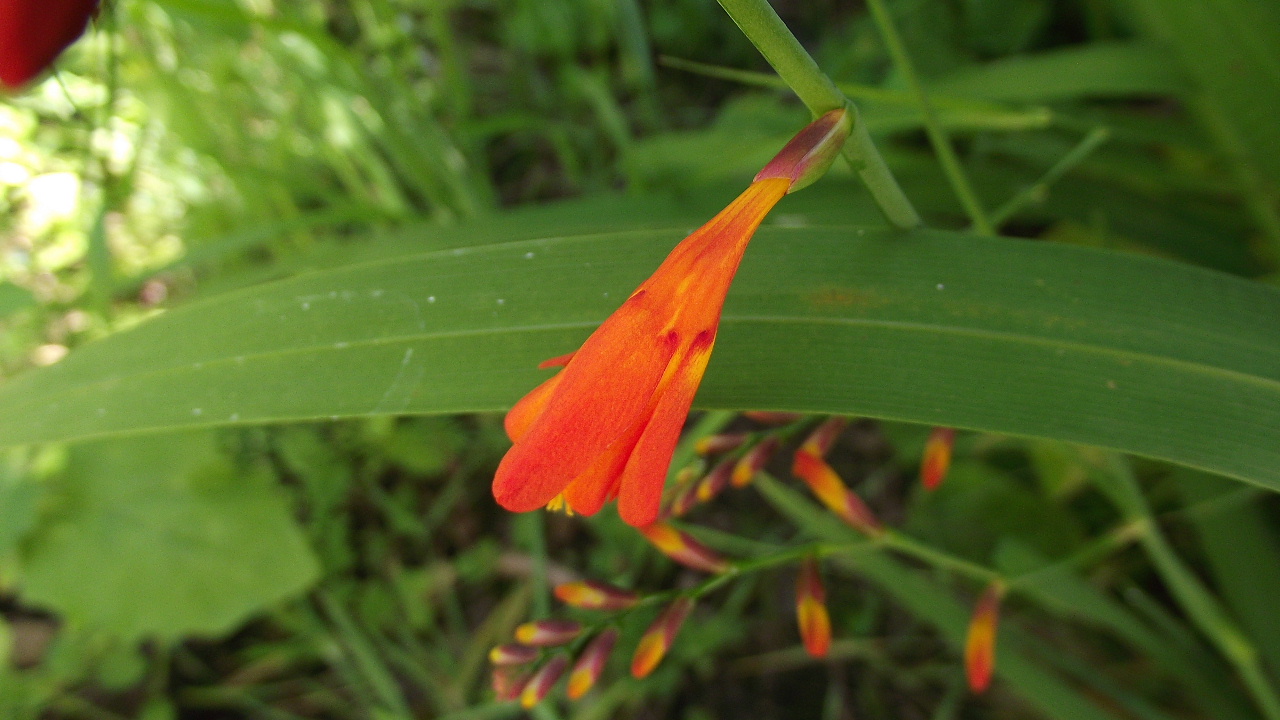This photograph captures a vibrant scene of dense vegetation in a natural setting. Dominating the foreground is a gracefully arcing blade of grass that stretches from the left side of the image to the right. Situated atop a prominent green stem, a small flower in the early stages of blooming stands out as the most in-focus element. This flower's petals exhibit a striking combination of orange, yellow, and a touch of purple near the base where they connect to the stem. Behind this main flower, the background is artistically blurred, highlighting the photograph's depth of field and revealing a mix of additional tall grasses, leaves, and another stem adorned with multiple closed flower buds of similar color. The overall composition exudes a palette of lush greens interspersed with bursts of vibrant orange, yellow, and hints of purple, creating a natural tableau that is both detailed and captivating.